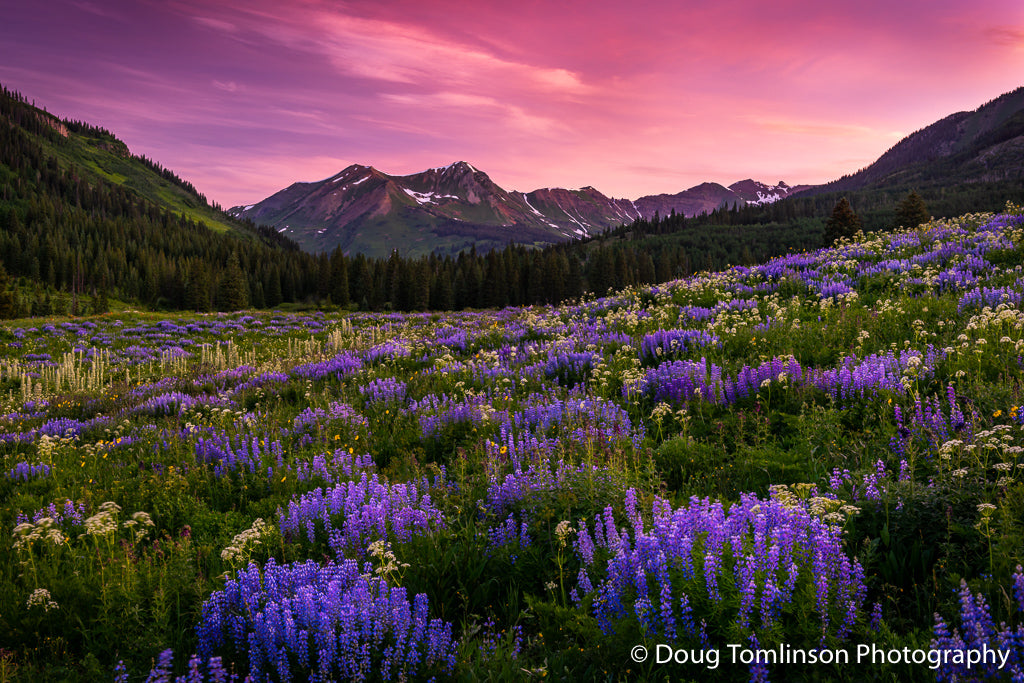This vibrant, highly detailed professional photograph by Doug Tomlinson captures a breathtaking field of flowers set against a scenic mountainous backdrop. Foremost in the image are clusters of bright purple flowers interspersed with smaller bunches of yellow blooms and a row of taller yellow flowers slightly left of center. Delicate white flowers lace the meadow, adding to its diverse beauty. The lower right corner of the image bears a copyright mark and the name "Doug Tomlinson Photography."

In the mid-ground, a lush row of pine trees lines the horizon, thicker on the left and gradually thinning toward the center before tapering off just before the right edge. These trees sit atop gentle hills framing the sides of the image. Between these hills lies a small mountain range characterized by a green base, rocky summits, and a light dusting of snow.

Above, the sky is a mesmerizing palette of purple, pink, and yellow hues, indicating the time is either at dusk or dawn. The clouds meld these colors in a harmonious display that illuminates the mountains beneath with a warm glow. The photograph, taken with what appears to be a wide-angle lens, is rich in color and detail, capturing the essence of springtime in a mountainous meadow bathed in the soft light of sunset.